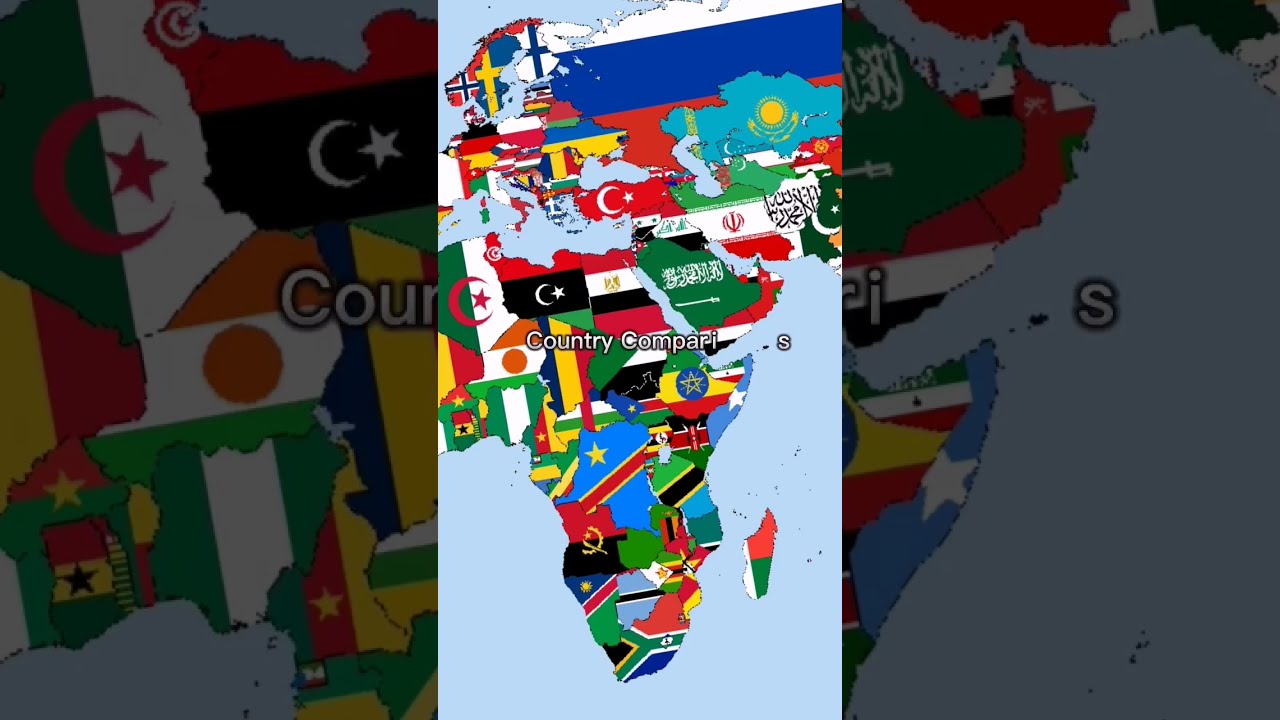This image is a composite map with a unique and detailed presentation. At the center, there's a vibrant map highlighting various countries, each delineated with its respective flag. The prominent colors on the map include blue, yellow, white, red, green, and black. The central part of the map displays the country of Mexico, although it does not follow a traditional cartographic design. Instead, the regions within this map are demarcated using an array of distinct symbols such as stars and banners, with some symbols resembling the letter 'C' with a star in the center.

Surrounding this main map, the image is split into three sections. On the far left and far right sides, darkened and enlarged segments of the center map are displayed, providing a zoomed-in view that emphasizes the details of specific regions. The background features a darker, more subdued hue of the central map, creating a layered, aesthetically appealing effect.

In the center of the map, the text "country Campari" is prominently written in white letters with a black outline. To the right of this text, the solitary letter "S" is spaced out, adding a unique textual element to the composition.